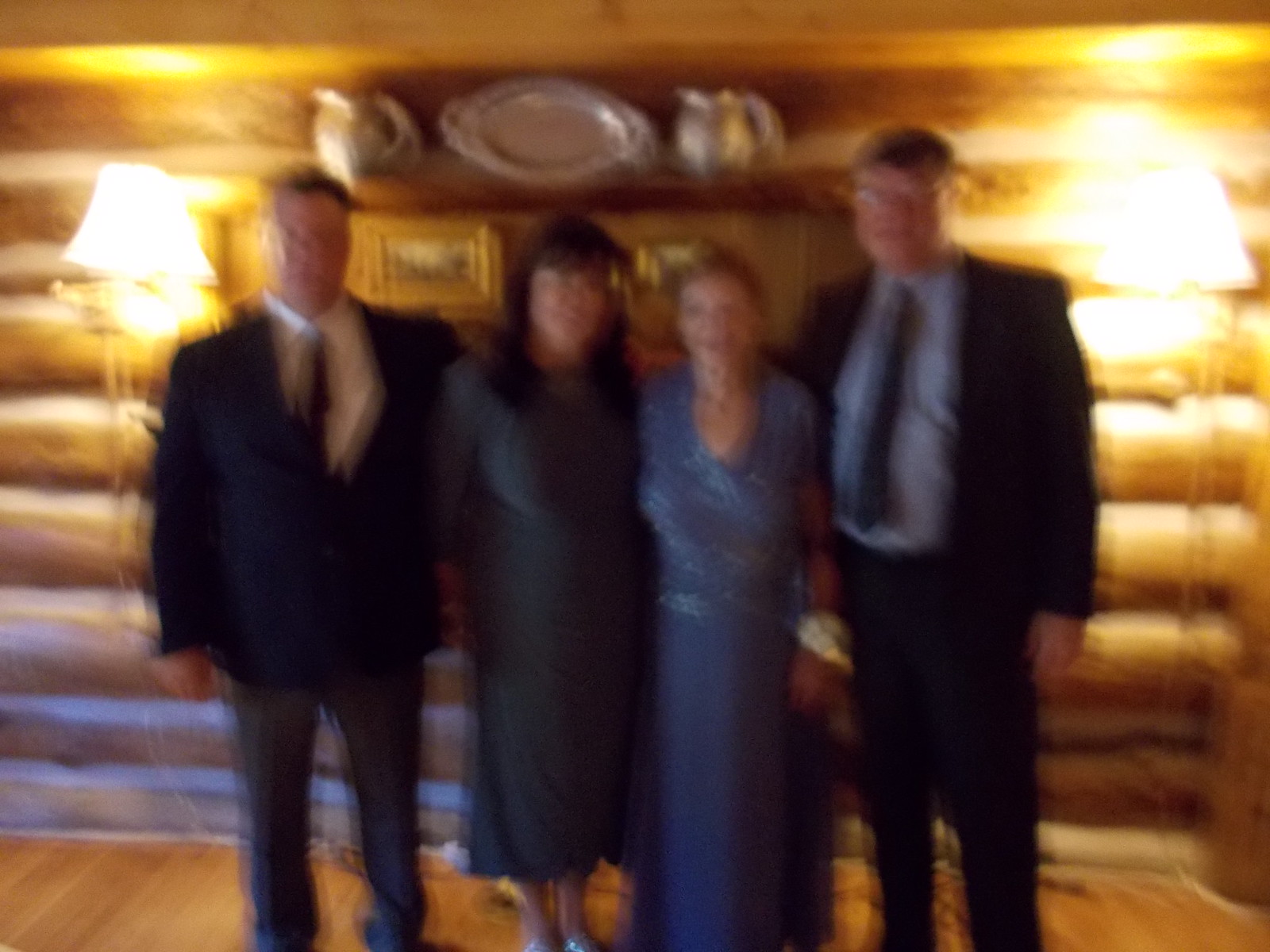This photograph captures four individuals standing in front of a rustic log cabin wall. The image is slightly blurry, affecting the visibility of detailed features. On the far right stands a man wearing a dark blue suit jacket and matching pants, paired with a blue tie and a light blue shirt. He has short brown hair, wears glasses, and he is positioned next to a woman in a blue dress adorned with a gold fabric draped around her left wrist. To her left is another woman dressed in a gray dress. The fourth individual, a man, stands farthest to the left. He is dressed in a navy-colored jacket with a white shirt and what appears to be a red tie, complemented by gray pants. The wooden log cabin wall behind them adds a charming, rustic backdrop to their formal attire.